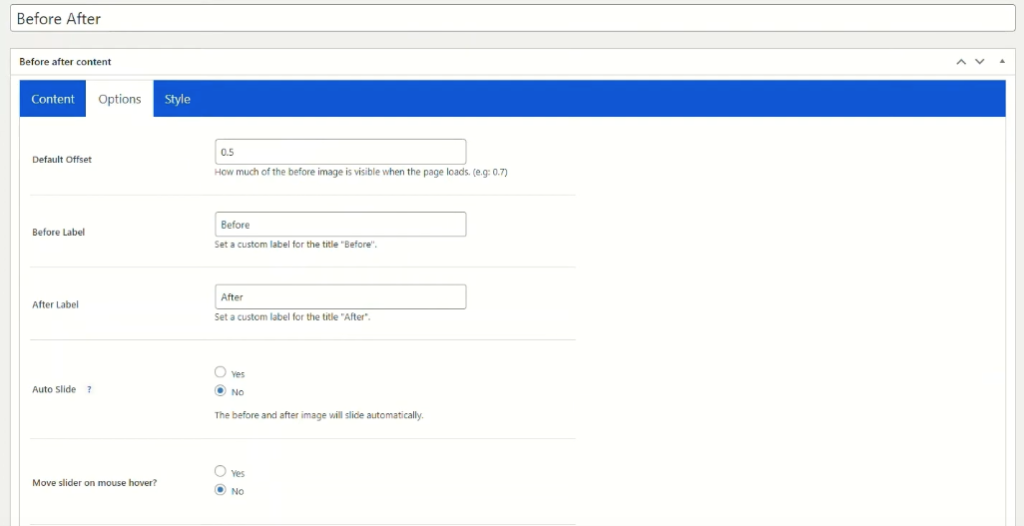The image depicts a web page interface designed for configuring a "before and after" comparison slider. At the top, there's a header labeled "Before After," followed by subheaders "Content," "Options," and "Style." Both "Content" and "Style" are highlighted with a blue background, while "Options" remains white, indicating it is the currently selected section.

In the "Options" section, there are several fields for customization:

1. **Default Offset**: Set at "0.5," with a description below explaining this controls how much of the "before" image is visible when the page loads, providing an example value of "0.7."

2. **Before Label**: Contains a text box with the default label "Before," allowing users to set a custom label for the "before" image.

3. **After Label**: Similar to the previous field, this text box has the default label "After," enabling customization of the label for the "after" image.

4. **Auto Slide**: This field offers a "Yes/No" option for automatically sliding the before and after images, with "No" currently selected. 

5. **Move Slider on Mouse Hover**: Another "Yes/No" option that determines if the slider should move when the mouse hovers over it; "No" is selected by default.

The interface also includes buttons featuring gray upward-facing and downward-facing arrows, numerous text boxes with white backgrounds, and gray accents, all indicative of a typical web page designed for users to customize various settings.